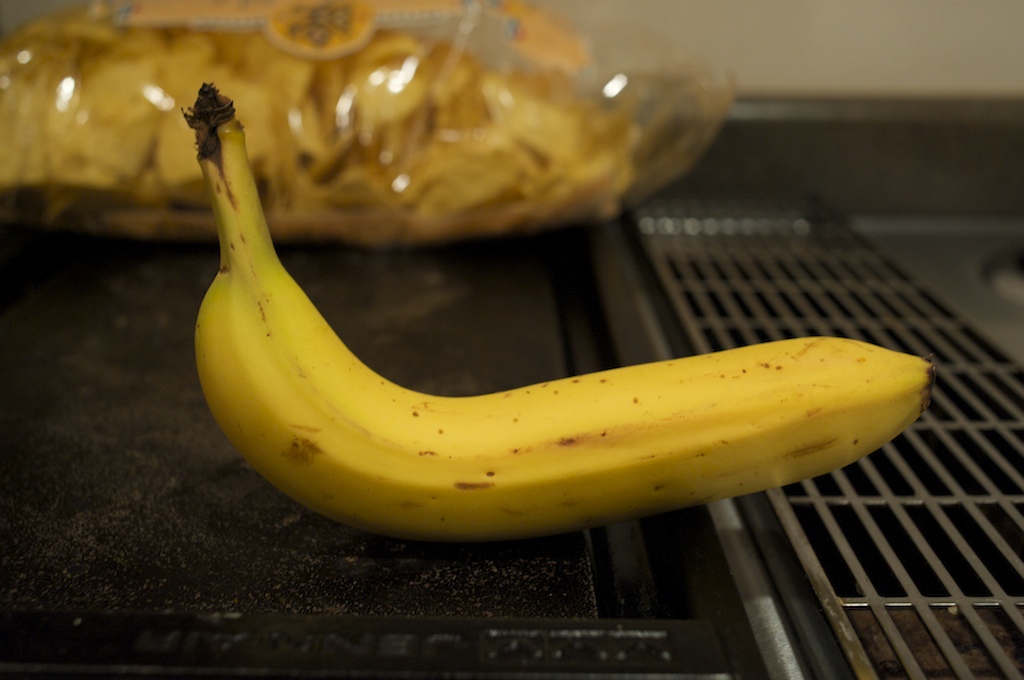The image depicts a single yellow banana with a few small browning spots, resting on a grill-like surface, possibly a stove or a cast iron counter. The banana is twisted off from the rest of its bunch. In the background, a blurry, closed plastic bag of chips can be seen. On the right side of the image, there's a stainless steel surface adjacent to the grill-like area. The surface the banana is on appears to have some upside-down and blurry lettering that is difficult to decipher. The scene is set in a kitchen environment with various textures and materials, including iron and steel.